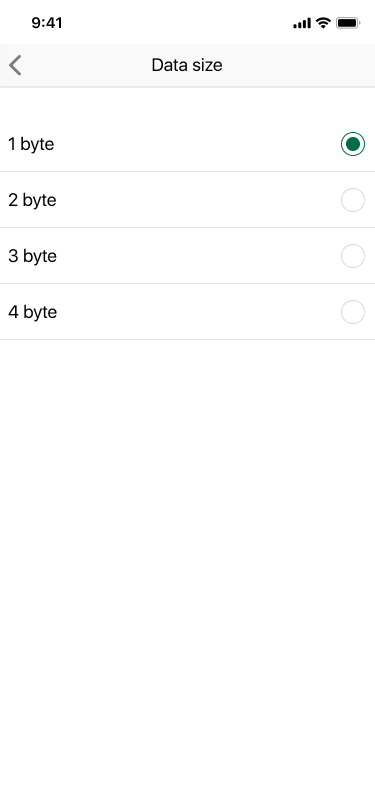The screenshot displays an iPhone interface, indicated by the 9:41 AM time at the top-left corner, alongside icons showing a strong cellular connection, active Wi-Fi, and an almost full battery. At the top of the screen, a header reads "Data Size," accompanied by a left arrow, suggesting a back button. Below the header, a selection menu with four options is present: "One Byte" (selected and highlighted with a filled green circle), "Two Byte," "Three Byte," and "Four Byte" (all unselected). The background is predominantly white, embodying Apple's signature clean and minimalist design. Despite the unclear context of "data size," the interface suggests a focus on small-scale data selection.